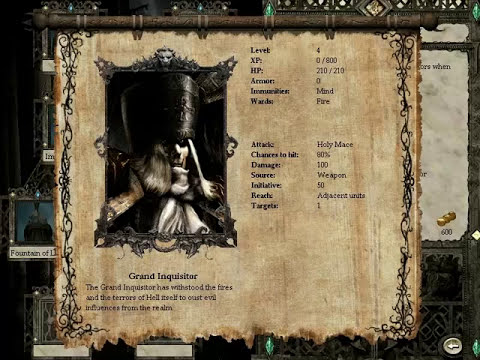The image depicts a detailed screenshot from a video game featuring an old, parchment-like scroll hung from a horizontal, round post. The main focus of the scroll is a rectangular framed image of a sinister-looking man named the Grand Inquisitor. He wears a tall black hat adorned with two furry parts covering his ears. His eyes are shadowed, and long hair cascades from beneath the hat, partially obscuring his face. He dons a white shirt and a black coat with a frilly front, reminiscent of the Victorian era, or perhaps even medieval times given the cross on his hat. Beneath the image, in small, black text, the scroll reads, "Grand Inquisitor: The Grand Inquisitor has withstood the fires and the terrors of hell itself to oust evil influences from the realm."

To the right of the image and text, the scroll displays various game statistics in small, difficult-to-read font: "Level 4," "XP 0 / 800," "HP 210 / 210," "Armor 0." Additional stats, including "Immunities: mind wards, fire," "Attack: holy mace," "Chances to hit: 80%," "Damage: 100," "Source: weapon," "Initiative: 50," "Reach: adjacent units," and "Targets: one," are also present, indicating the character's specific abilities and attributes within the game.